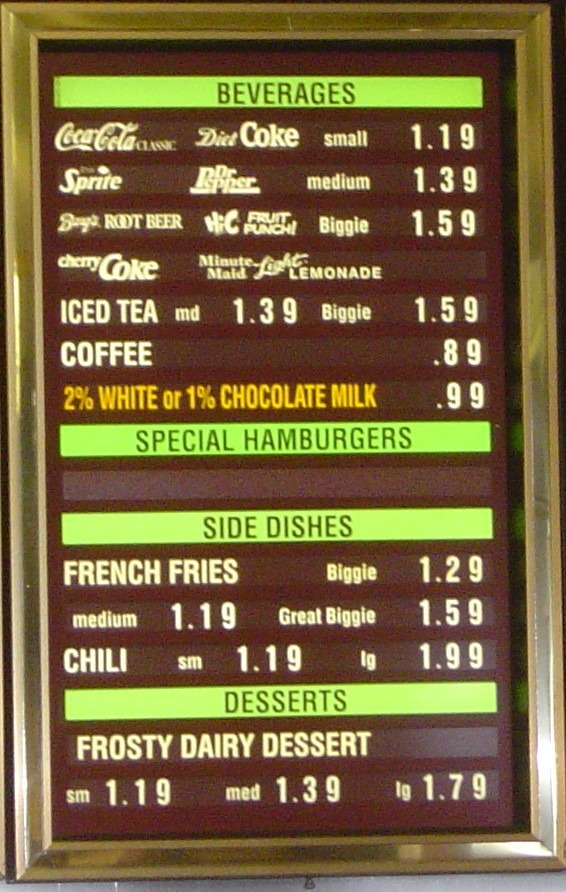This close-up photo depicts a vintage Wendy's menu encased in an ornate gold frame. The menu itself features a rich brown background with green category headers adorned with brown lettering. The top category, "Beverages," details various drink options along with their sizes and prices. Beneath this, a section titled "Special Hamburgers" appears, although no items are listed under it. The third category, "Side Dishes," enumerates items like french fries and chili along with their respective prices. At the bottom, the "Desserts" section lists Frosty options, specifying prices for small, medium, and large sizes. Below the menu, part of a white wall is visible, while a dark shadow encroaches from the top right corner beside the menu, extending down to the bottom left where it becomes particularly intense and black. Notably, all menu items are printed in white letters except for the 2% white or 1% chocolate milk, which is highlighted in yellow.